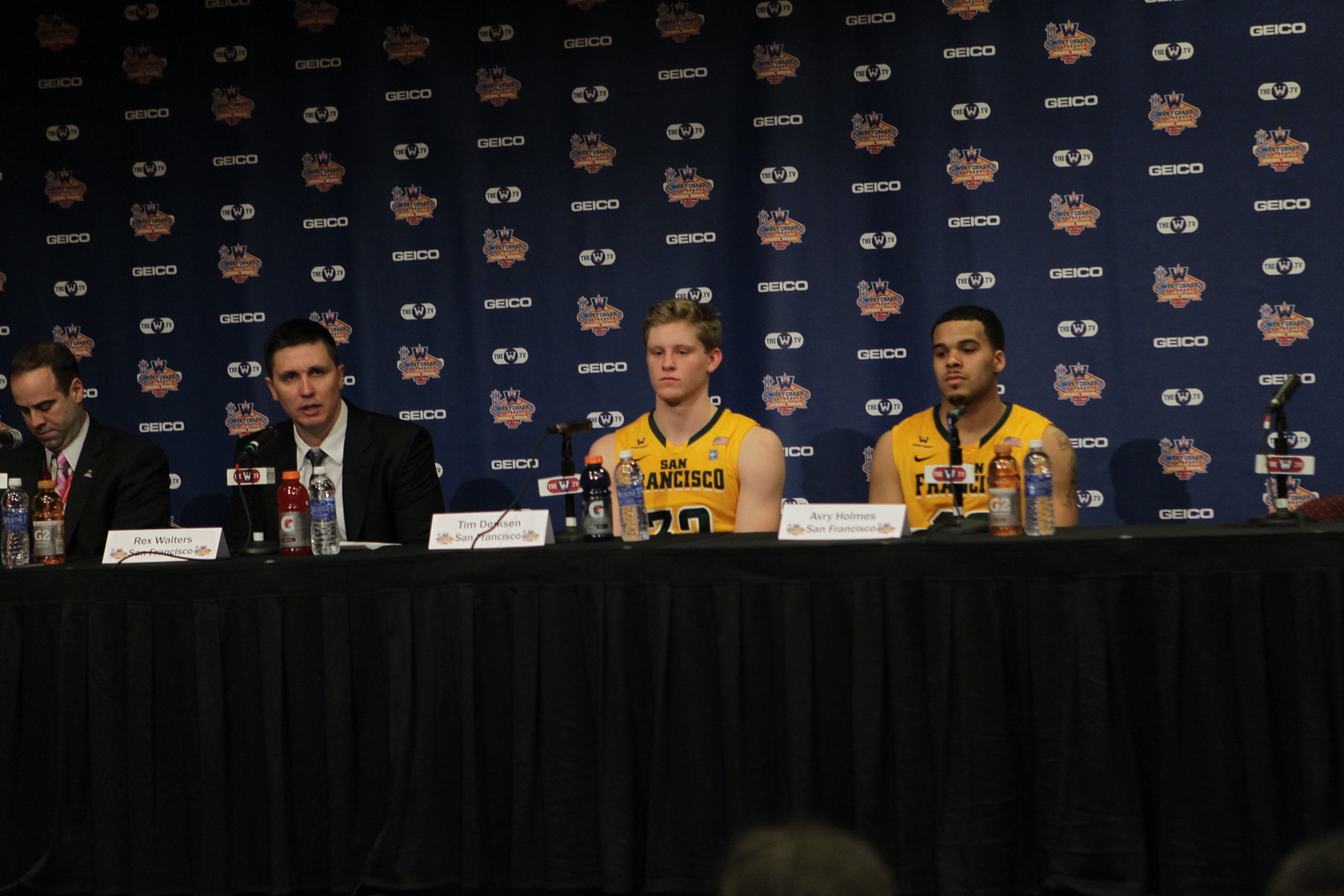This image captures a post-game sports conference set in a room with a long table covered in a dark cloth. Four men are seated at the table, which is positioned in the center of the image. In front of each man, there are Gatorade bottles and water, along with microphones, indicating they are about to speak or just have spoken. 

From left to right: the first man is in a suit and tie, looking downward. The second man, also in a suit and white shirt, has his tent card labeled "Rex Walter San Francisco." The third man is wearing a yellow basketball jersey with black numbering that reads "San Francisco," and his tent card says "Tim Dirksen San Francisco." The last man on the right, also in a yellow "San Francisco" jersey, appears downcast, with his tent card reading "Avery Holmes San Francisco." 

In the backdrop, multiple advertisements are visible, including for Geico and likely "West Coast," contributing to a professional and branded atmosphere typical of sports press conferences. The colors present in the scene include black, yellow, blue, white, dark blue, brown, orange, and purple, enriching the image's overall vibrancy.